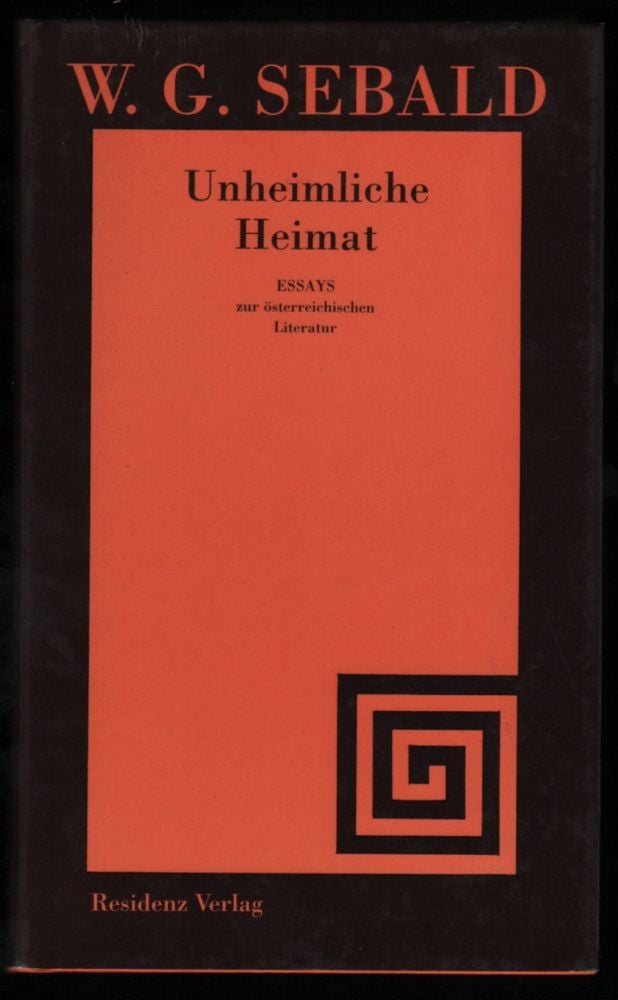This is a photograph of the front cover of a book. The background is predominantly black with a large red rectangle at its center. Within this red rectangle, at the top, is the author's name in red text: "W.G. Sebald" (S-E-B-A-L-D). Beneath the author's name, also in red, is the title in German: "Unheimliche Heimat" (U-N-H-E-I-M-L-I-C-H-E, H-E-I-M-A-T), followed by the word "Essays" in black, and further text in German: "zur Österreichischen Literatur" (Z-U-R, O-S-T-E-R-R-E-I-C-H-I-S-C-H-E-N, L-I-T-E-R-A-T-U-R). At the bottom right corner of the red rectangle, there is a detailed black spiraling feature that looks like a square pattern getting smaller and smaller. At the very bottom of the cover, the publisher's name is displayed: "Residenz Verlag" (R-E-S-I-D-E-N-Z-V-E-R-L-A-G).